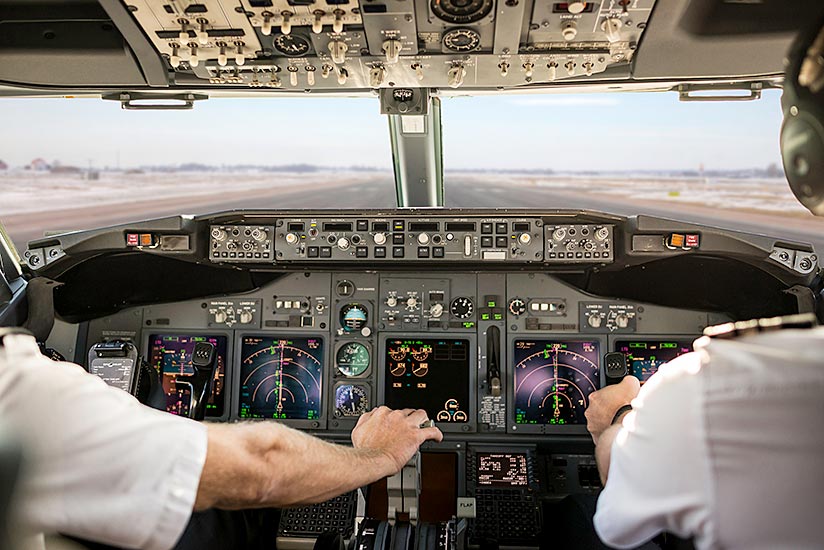The image captures an interior view of a jumbo jet cockpit from a perspective just behind the two pilots’ seats. Both pilots, dressed in white short-sleeved shirts with emblems on their shoulders and with headsets on, are engaged in their pre-flight procedures. The pilot on the left is extending his right arm forward, seemingly grasping a throttle lever, while the pilot on the right holds a control stick with both hands. The cockpit is dominated by an impressive array of instrumentation, including dials, gauges, radar screens, buttons, switches, and overhead panels filled with more controls. Through the narrow cockpit windows, the runway stretches out ahead, slightly blurry, suggesting the aircraft is positioned and ready for takeoff. The outside scene appears desolate, possibly a desert or snow-dusted prairie, and the clear daytime sky promises favorable flying conditions. The image may be a computer-generated graphic, though the intricate details of the controls and the pilots' focused postures add a layer of realism.